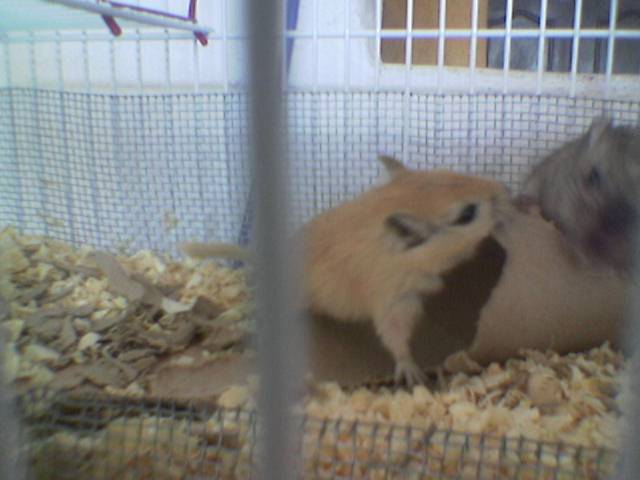This grainy photograph captures the inside of a hamster cage, showcasing two hamsters interacting with one another. The beige hamster, situated in the middle and looking towards the gray hamster, is sniffing or closely facing the gray hamster, which gazes directly at the camera. The hamsters appear to be standing on a partially chewed toilet paper roll, which acts as a playful tunnel. The cage floor is covered with light tan wooden shavings or cardboard flakes, along with darker scraps of the chewed toilet paper roll. The white bars of the cage, along with some mesh or netting material, are visible in the background, framing the well-maintained and healthy-looking hamsters.